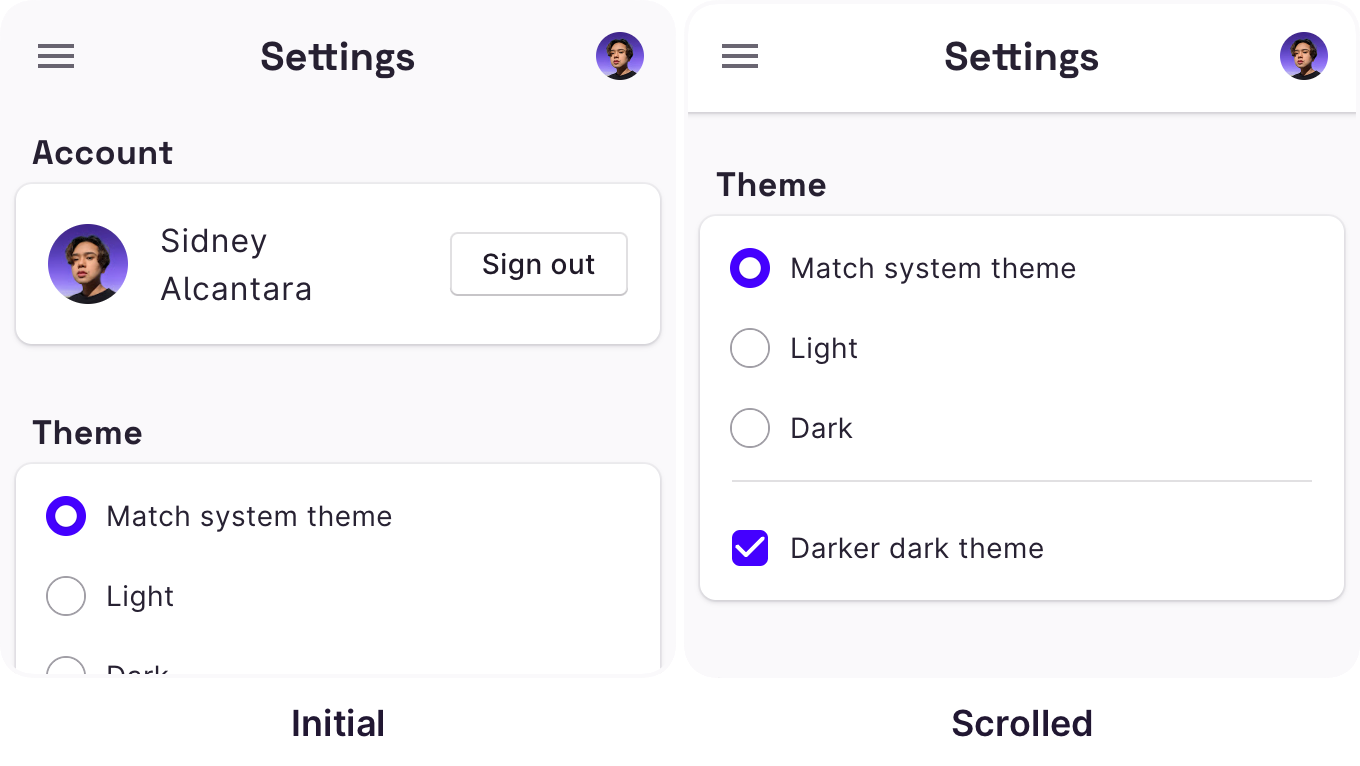The image consists of two side-by-side screenshots depicting settings menus for a software application. 

In the left screenshot:
- The background is green with three horizontal lines located in the upper left corner, indicating a menu icon.
- The screen is titled "Settings" and features an image of a person with a metrosexual appearance, characterized by a darker skin tone, black hair, and an edgy style, wearing a black t-shirt.
- Below the image, the word "Account" is displayed, followed by a pop-up window with a white background. The window contains the person's name, "Sidney Anclair" (possibly Spanish).
- A black button labeled "Sign Out" is situated below the name.
- Further down on the gray background, the section titled "Theme" appears. A white box lists the options: "Match System Theme," "Light," and "Dark," each accompanied by a gray circle on the left. The "Match System Theme" option is highlighted in blue.
- The section is concluded with the word "Initial" in black at the bottom.

In the right screenshot:
- The layout is similar, but the settings section is surrounded by a white background.
- The same "Theme" options are presented, showing the "Dark" theme selected, indicated by a blue square with a white check mark and the text "Darker dark theme has been selected" in black.
- The interface is awaiting user interaction, as indicated by the white check mark highlighting the active selection.